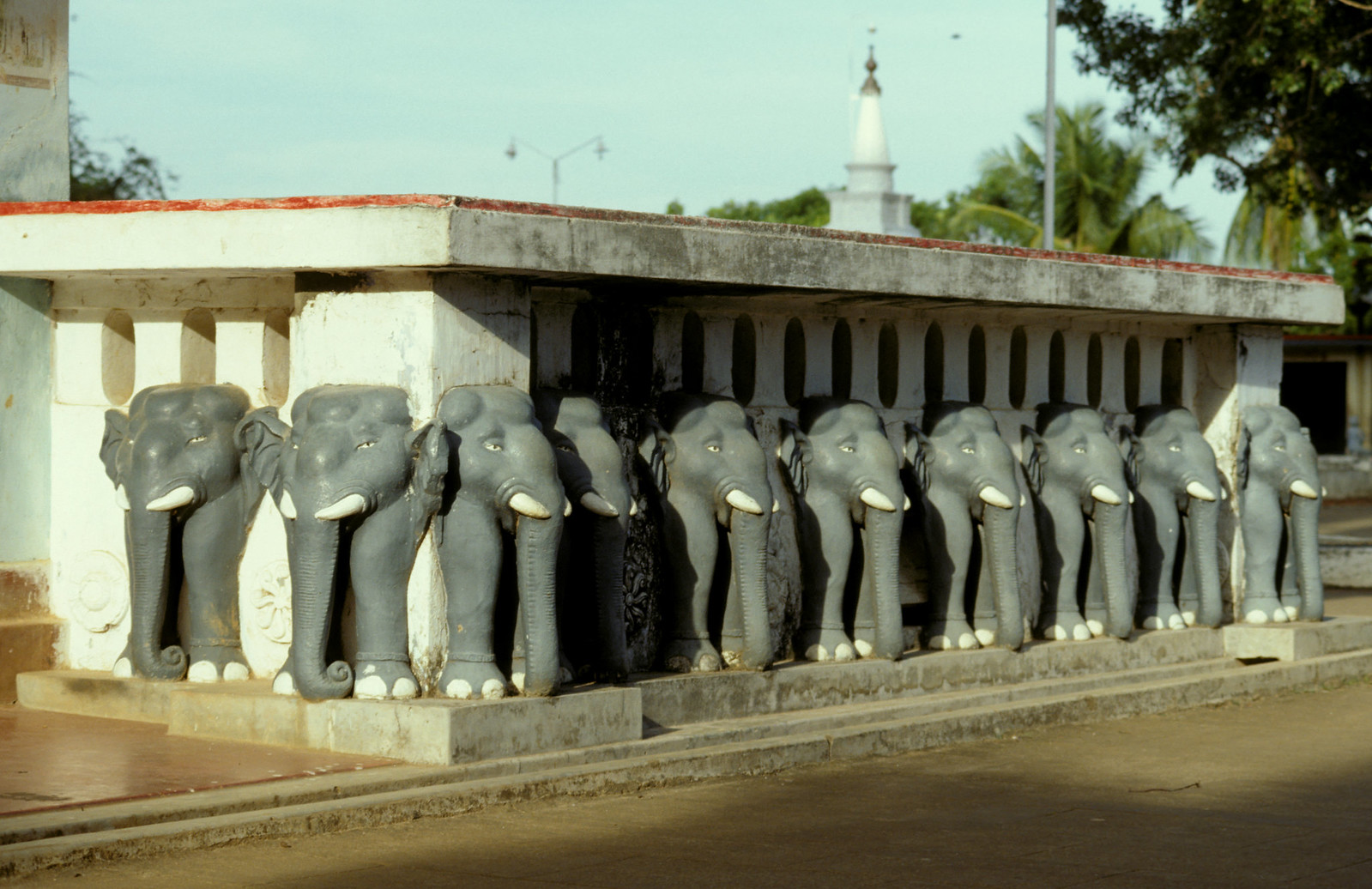The image depicts a small, white, rectangular building with a somewhat worn, flat red roof, highlighted by a sliver of red tint. The building's exterior is adorned with gray elephant statues, with only their front halves visible, seemingly emerging from the structure. Each elephant has distinct white tusks, eyes, and toenails. Alongside the building, the elephants' heads, trunks, and forelegs are seen, with the trunks curling gracefully under their feet. These statues form a line, with two on the left side and eight at the front. In between the elephants are additional bas-reliefs of floral designs, crafted in the same white hue as the building.

The building appears to be mounted on a raised gray concrete platform, bordered by a concrete curb and intersected by a mix of brick walkways and concrete pavements. The surrounding area includes a dirt road turning to mud, suggesting a well-used pathway. The landscape features a few scattered trees and streetlights, while the background reveals a tall, steeple-like structure and palm trees against a light blue sky. Despite its illustrative and somewhat surreal presentation, the scene's architectural and cultural elements suggest a possible location in India.